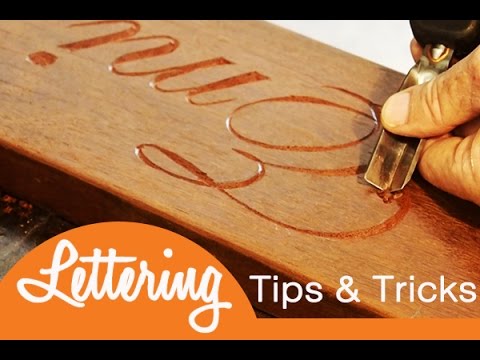This image showcases a scene from what appears to be a YouTube tutorial titled "Lettering Tips and Tricks," as indicated by white cursive text within an orange half-circle at the lower part of the image. The bottom black border further emphasizes the title. The focal point of the image is a person's hand meticulously carving cursive letters into a piece of wood using a pointed metal tool, possibly a rotary or burning tool. The person's fingers and the tool are clearly visible on the right side of the image, while the carved letters are prominently displayed on the left. The background is solid white, making the wooden board and the hand-carving activity stand out. The scene is set indoors, encapsulating a detailed moment of craftsmanship and instructional guidance.